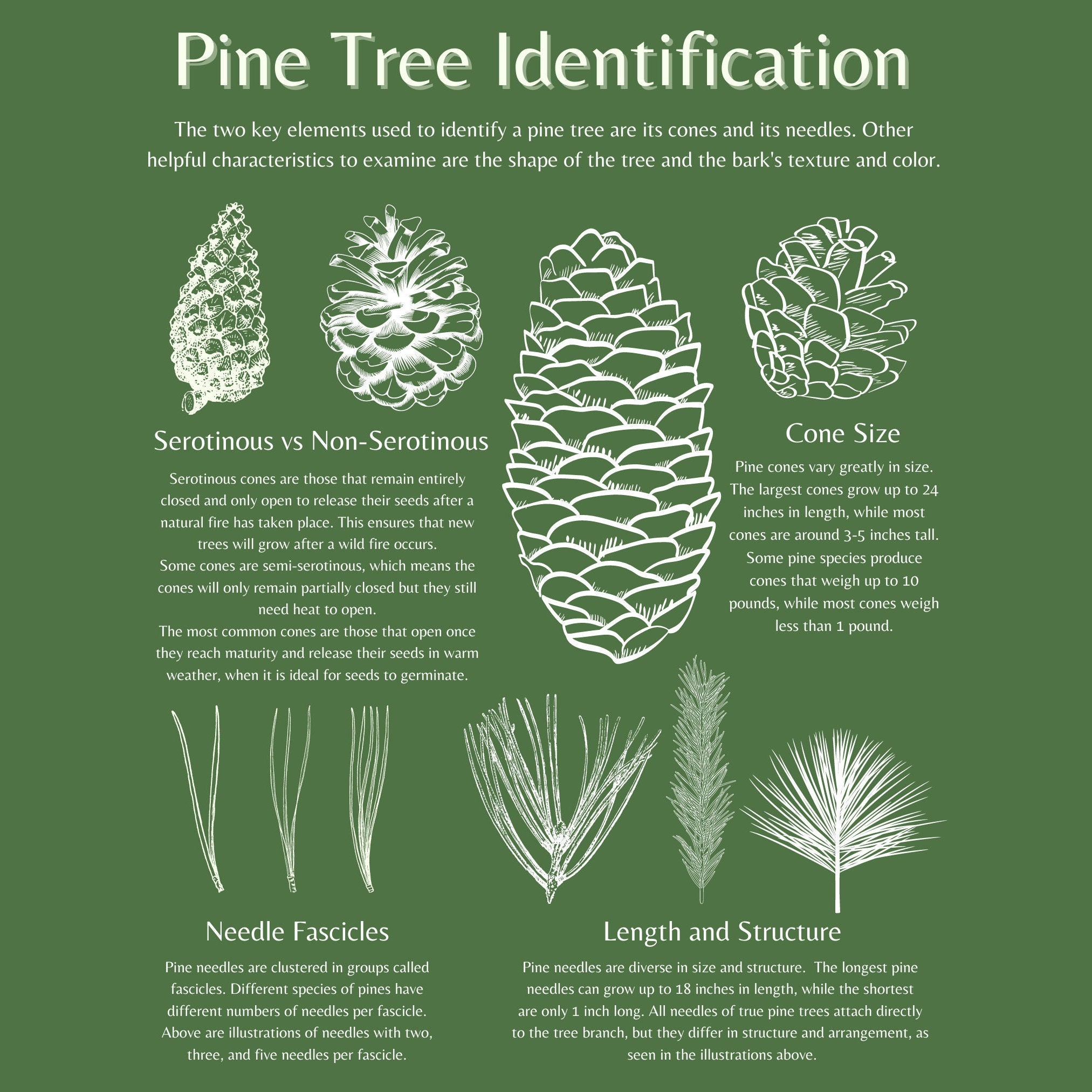This square banner features a forest green background adorned with white text and illustrations dedicated to "Pine Tree Identification." At the top, large text emphasizes that the two key elements for identifying a pine tree are its cones and needles. Additional characteristics to consider include the tree's shape and the bark's texture and color. Below this text, there are four detailed white illustrations of pine cones. On the left side, an article titled "Serotinous versus Non-Serotinous" discusses different types of cones, with illustrations above and detailed text below. To the right, another section titled "Cone Size" explains that pine cones vary significantly in size, with the largest reaching up to 24 inches in length and some weighing up to 10 pounds, although most are 3 to 5 inches long and weigh less than 1 pound. The bottom left corner titled "Needle Fascicles" displays three illustrations of pine needles, while the bottom right corner, labeled "Length and Structure," details the length and formation of the needles.